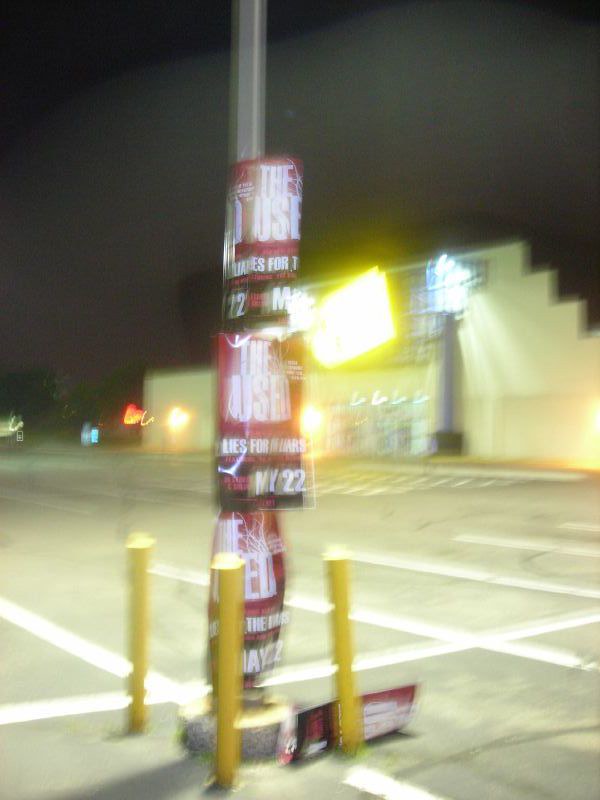A vertical nighttime color photograph captures a hazy, dimly lit parking lot bathed in a yellowish glow from street lighting. White lines traverse the light gray asphalt, denoting parking spaces. Central in the image, a metal pole with a cement base is adorned with black, white, and red banners or flags, though their precise nature is obscured due to the blurriness. Surrounding the base are three yellow cement posts. In the background, a building with a stair-stepped edge looms, partially illuminated by a bright light that might be on or near it. The rest of the scene dissolves into a murky, black sky, contributing to the overall blur of the photograph.